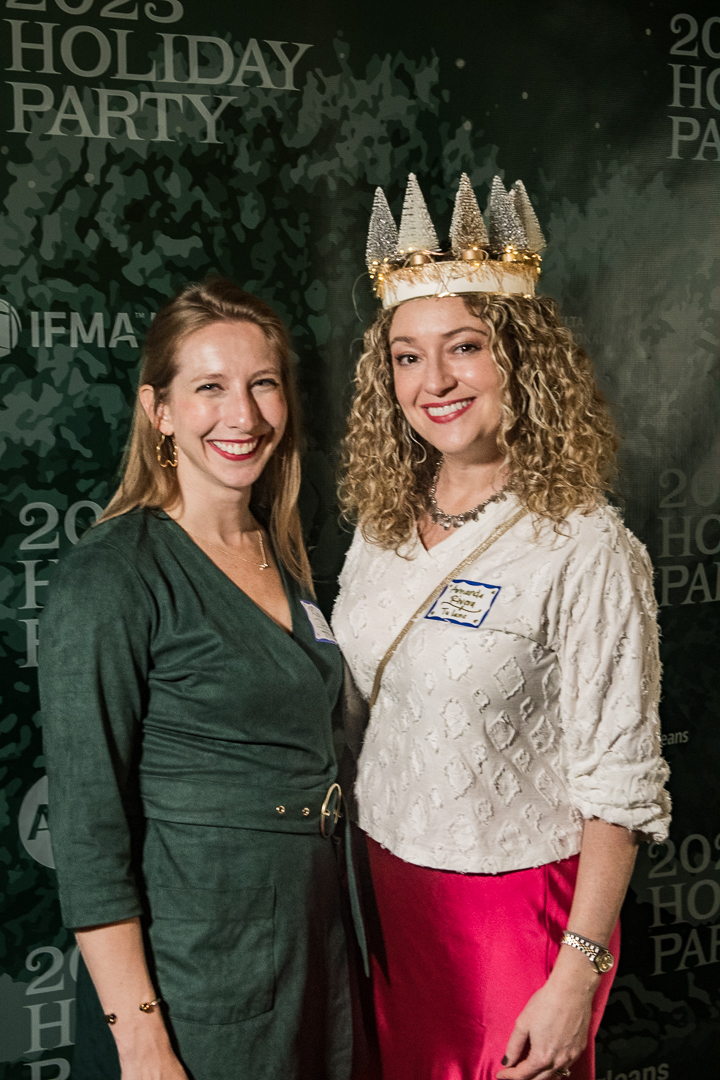In this vibrant holiday-themed photo, two young women stand shoulder to shoulder, smiling brightly. Both women wear red lipstick, adding a festive touch to their appearances. The woman on the left, with long, straight honey blonde hair, is dressed in a dark green dress cinched with a golden belt and accessorized with a bracelet on her right arm. Her massive smile exudes joy and warmth. Standing close to her is a woman with curly, shoulder-length blonde hair, adorned with a crown featuring white Christmas trees and lights. She is dressed in a white blouse paired with a shiny red skirt and a golden watch on her left wrist. Behind them is a green wall emblazoned with the words "Holiday Party," alongside various sponsor logos. The background is festively adorned, contributing to the celebratory atmosphere of the event.